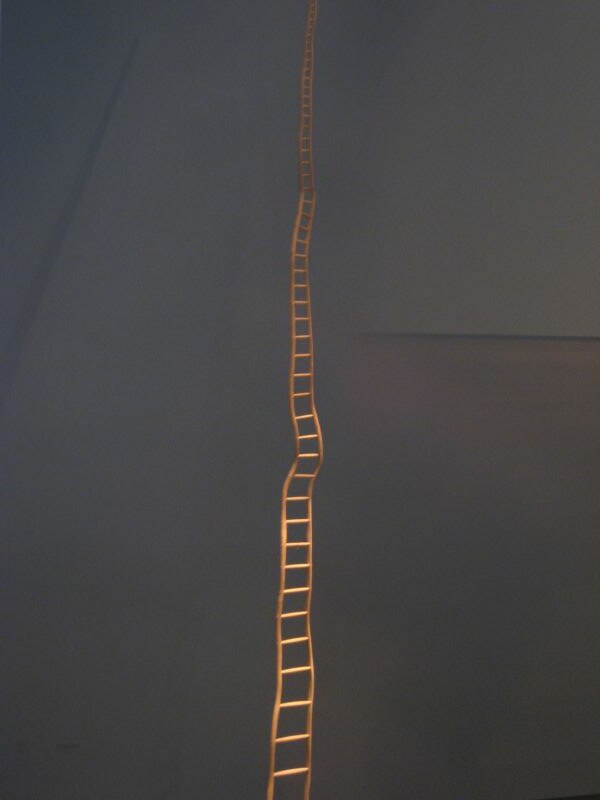This image, possibly an art installation or computer-generated, features a thin, irregularly shaped bronze ladder extending dramatically upwards into the sky. The ladder, with a color described variously as bronzy golden brown and yellow goldish, stands out vividly against a backdrop that shifts in hues from dark blue to a night-like black-gray. The background has a surreal quality, adding to the elusive nature of the scene.

The ladder itself begins larger at the bottom and narrows as it ascends, warping with waves and curves as if affected by underwater refraction. It features golden cylinders or pipes connecting the two sides, creating steps and handholds. The structure bends and twists to the right and left at various points, adding to its mystical, almost otherworldly appearance. Light reflects off its surface in places, accentuating its metallic sheen, while the backdrop maintains a mysterious, dreamlike atmosphere. The higher sections of the ladder fade into darkness, enhancing the impression of infinite ascent.